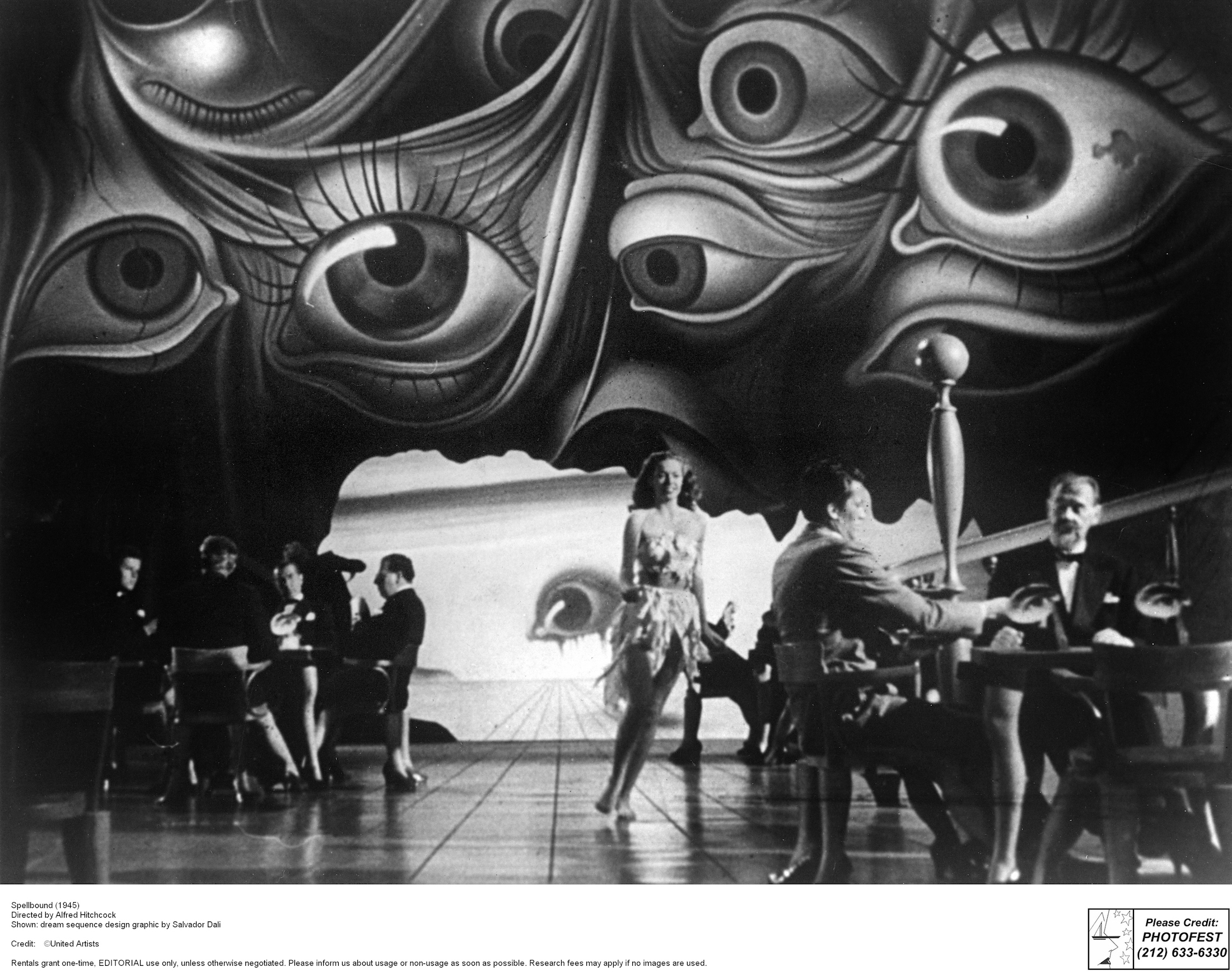This detailed black and white photograph from the 1945 Alfred Hitchcock film "Spellbound" captures an abstract dream sequence designed by Salvador Dali. The scene, intended for editorial use, features a surreal restaurant setting with large, pronounced eyeballs adorning the spooky ceiling. There are about ten irises, giving an eerie atmosphere to the room. In the center, a woman in a short dress walks barefoot towards seated men who are dressed in suits and ties. The dining tables are occupied by individuals engaged in conversation, both men and women, and there's a strange art piece—a ball on a tapered cylinder. The background of the image includes a painted mural that mirrors the restaurant with an additional eye. Below the photograph, a white border with black text provides a description, although the text is too small to be legible. The entire scene, rendered in shades of white, black, and gray, highlights the bizarre, dreamlike quality typical of Dali's artistic style.